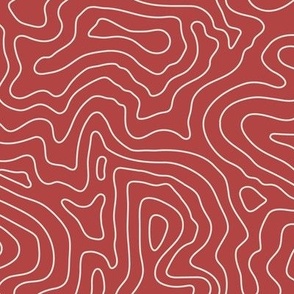This image showcases an abstract design with a maroonish-orange to brownish-red background, resembling a pastel blood-red hue. The composition is populated with thin, white squiggly lines, intricately sprawled across the canvas. These lines meander in a seemingly random fashion, evoking the look of topographic maps or elevation charts, yet they do not intersect. Amongst this intricate web of lines, some form irregular closed loops and circles, connecting in subtle and complex ways. The overall design, square in shape, bears a delicate, maze-like quality. Each line appears meticulously drawn, contributing to the intricate and captivating simplicity of the pattern.